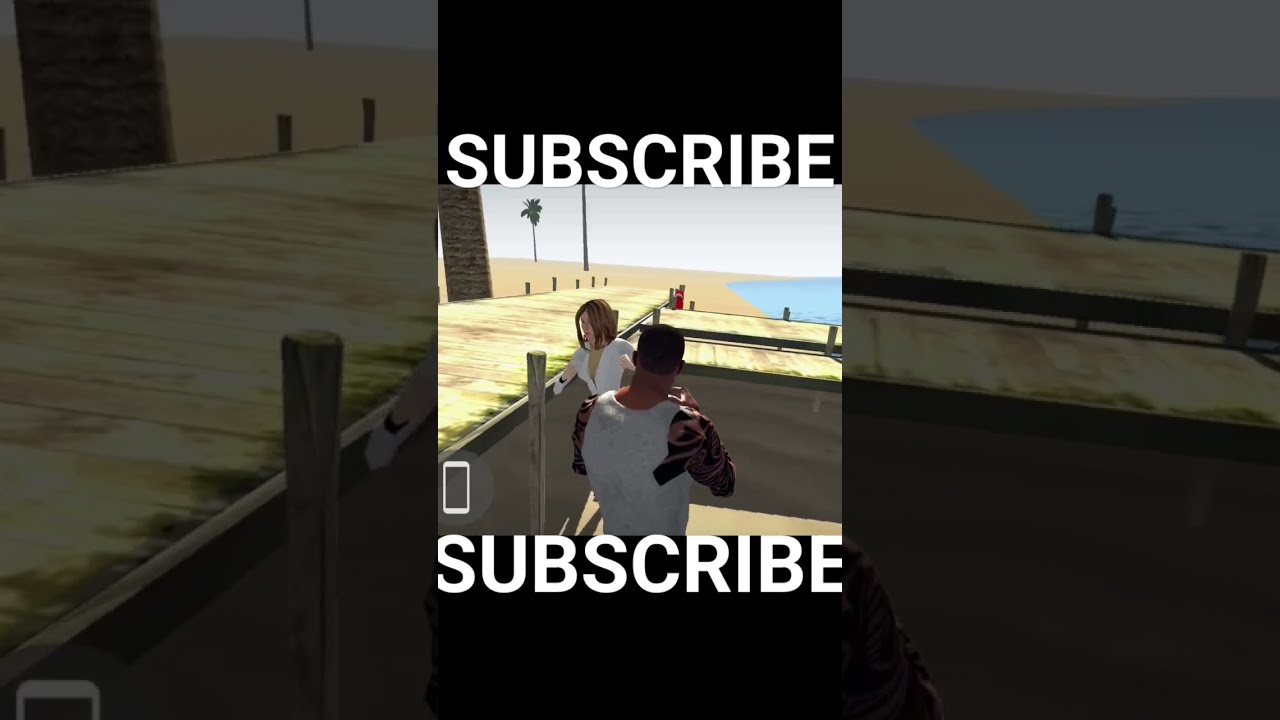The image depicts a screenshot from a video game being advertised on social media, possibly on YouTube, TikTok, or Instagram. The central focus is a man wearing a white tank top with black and white tattoos covering his arms, seen from behind. He stands on a beach, facing a woman in a white blouse with shoulder-length blonde hair. Surrounding them are palm trees, sand, water, and a wooden T-shaped dock extending into the sea. The image is overlaid on a dimly lit, horizontally stretched background of the same scene. Both the top and bottom of the image feature thick black bars with large, white capitalized text urging viewers to "SUBSCRIBE."